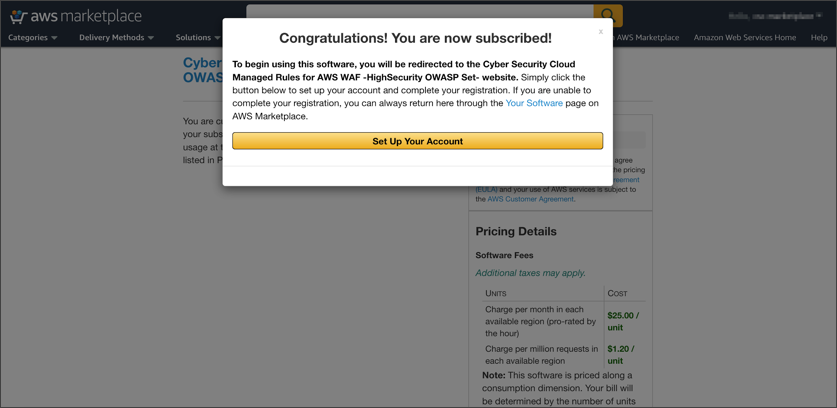The image depicts a greyed-out screen of AWS Marketplace. Superimposed over this screen is a prominent pop-up message, congratulating the user with the text: "Congratulations, you are now subscribed," written in black-colored font on a white background. Below this congratulatory message is a detailed paragraph providing further instructions. The text states: "To begin using this software, you will be redirected to the cybersecurity cloud to manage rules for AWS WIF-HIGHSECURITY OWASPSET-WEBSITE. Simply click the button below to set up your account and complete your registration. If you are unable to complete your registration, you can always return here through the Your Software page on AWS Marketplace." The words "Your Software" are printed in blue, indicating a hyperlink.

Beneath the instructional text, there is a distinct yellow button with the words "Set up your account" centered in black font. In the background, the greyed-out AWS Marketplace screen shows some pricing details for various listings.